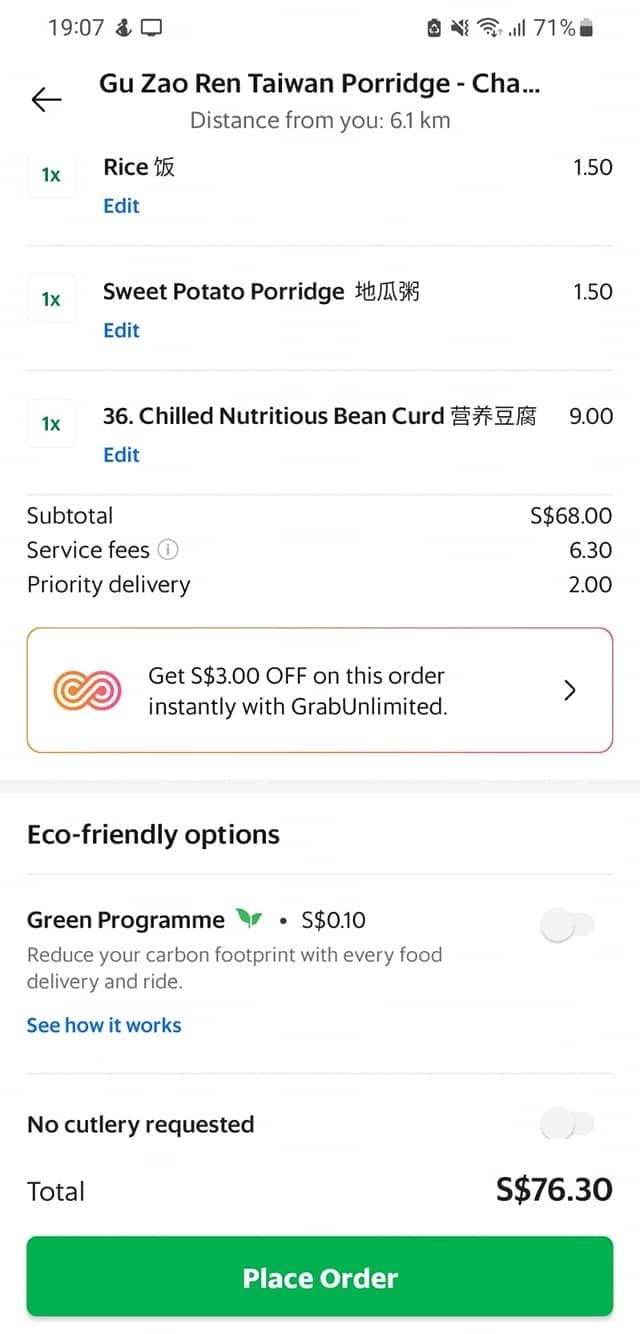### Detailed Caption for Shopping Screenshot:

The screenshot captures a user shopping on their cell phone, displayed against a white background.

**Top Section:**
- **Top Left Corner:** The time is shown.
- **Top Center:** The cellular signal strength, a Wi-Fi icon indicating full connectivity, and a muted sound icon. 
- **Top Right Corner:** The battery status, currently at 71% and charging.

**Header:**
- On the left, there's a black backward arrow.
- In bold black letters: "GUZ A0 Ren Taiwan Porridge - CHA..."
- Centered below the header: "Distance from you 6.1 kilometers."

**Main Content:**
- **Listed Items:** Displayed in black text with details about the number of times each has been purchased.
- **Edit Option:** In blue, offering the ability to modify items.
- **Cost:** Positioned on the right side.

**Summary Section:**
- **Subtotal, Service Fees, and Priority Delivery:** Listed with corresponding costs on the right.

**Promotional Pop-Up:**
- A white overlay featuring two red-bordered white infinity symbols.
- Text: "Get $3 off this order instantly with GrabUnlimited." Followed by a ">" symbol.

**Footer Section:**
- **Eco-Friendly Options:** Toggled off, it mentions a green program for $0.10 to reduce the carbon footprint with a link in blue: "See how it works."
- **No Cutlery Requested:** Toggled off in bold black text.
- **Total Cost:** $76.30.
- **Order Button:** Green tab with white text: "Place Order."

This organized view highlights all essential elements of the shopping interface, ensuring an intuitive and detailed user experience.